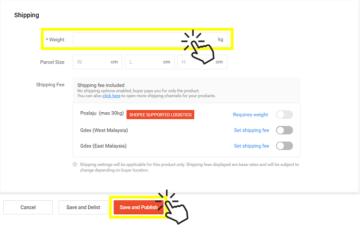The image depicts a detailed landing page for a logistics or e-commerce platform related to shipping and item dimensions. 

At the top left corner, against a white background, the word "Shopping" is displayed prominently in bold black font. Directly below, a yellow rectangular section includes labels for weights and measurements: on the left, it says "Weights," and on the right, "Kilograms (kg)." An illustrative finger icon with radiating lines indicates it’s clicking the search option for weight.

Further down, the page outlines dimensions: labeled "Potential Size," two side-by-side rectangles contain fields for "W (cm)" and "L (cm)." Another section reads "M (cm)" with associated input fields. 

Below these inputs, there’s a segment addressing shipping costs labeled "Shipping Fee." In a blurred grey rectangle, the phrase "Shipping Fee Included" can be discerned, accompanied by a legible "Click Here" hypertext link for further actions.

The page continues with a white rectangle housing various logistics options. Details are somewhat blurry, but it’s possible to make out entries like "POSLAJU (max 30 kg)." Adjacent to this is an orange rectangle with white text reading "Shop Pay Supported Linguistics." The term "Required Weight" appears next to a turned-off slider.

Additional entries include "GDEA (West Malaysia)," with a checkbox indicating "Set Up Shipping Fee" as active, and "GDEX (East Malaysia)," also labeled with a "Set Up Shipping Fee" checkbox that is turned off.

At the bottom of the page, three clickable buttons are visible: a white button with black text that says "Cancel," another button labeled "Save and Delist," and the final button highlighted with a hand symbol. This button has an orange background and white text reading "Save and Publish."